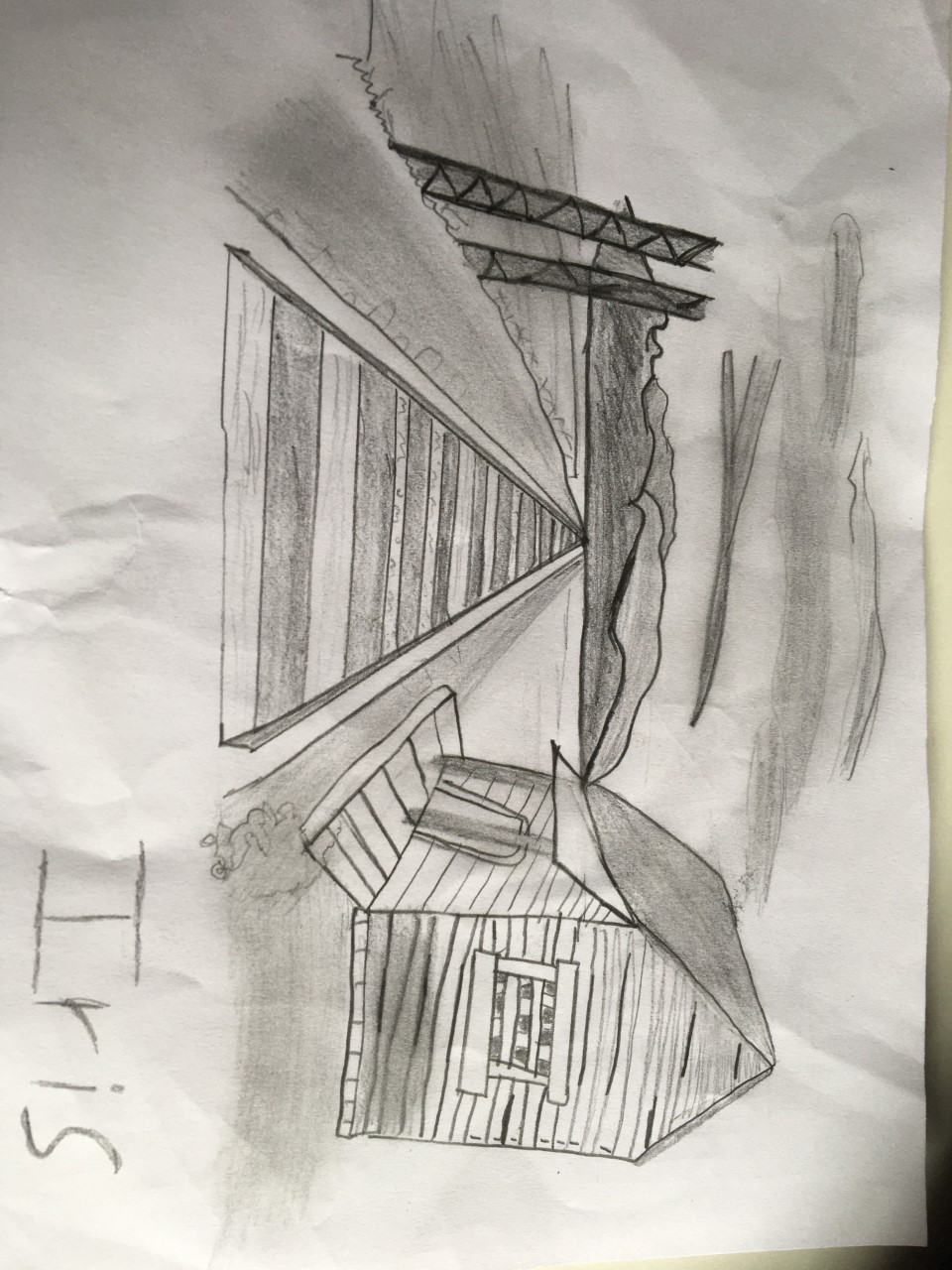This image depicts a slightly tilted black-and-white drawing on white paper, resembling an artistic sketch, signed by Iris in the right-hand corner. The focal point of the drawing is a wooden house situated on the right side, featuring a triangular roof, a single door, and one window. Extending from the house and running through the middle of the composition are railroad tracks, which guide the viewer's eye towards the background. In the distance, the scene transitions into rolling hills and mountains. On the left side of the tracks, there are numerous metallic beams and what appear to be tree-like structures. The sky above is filled with gray clouds, hinting at an impending rainstorm. The overall presentation of the drawing suggests it may have been casually stored and retrieved, adding to its raw and authentic charm.